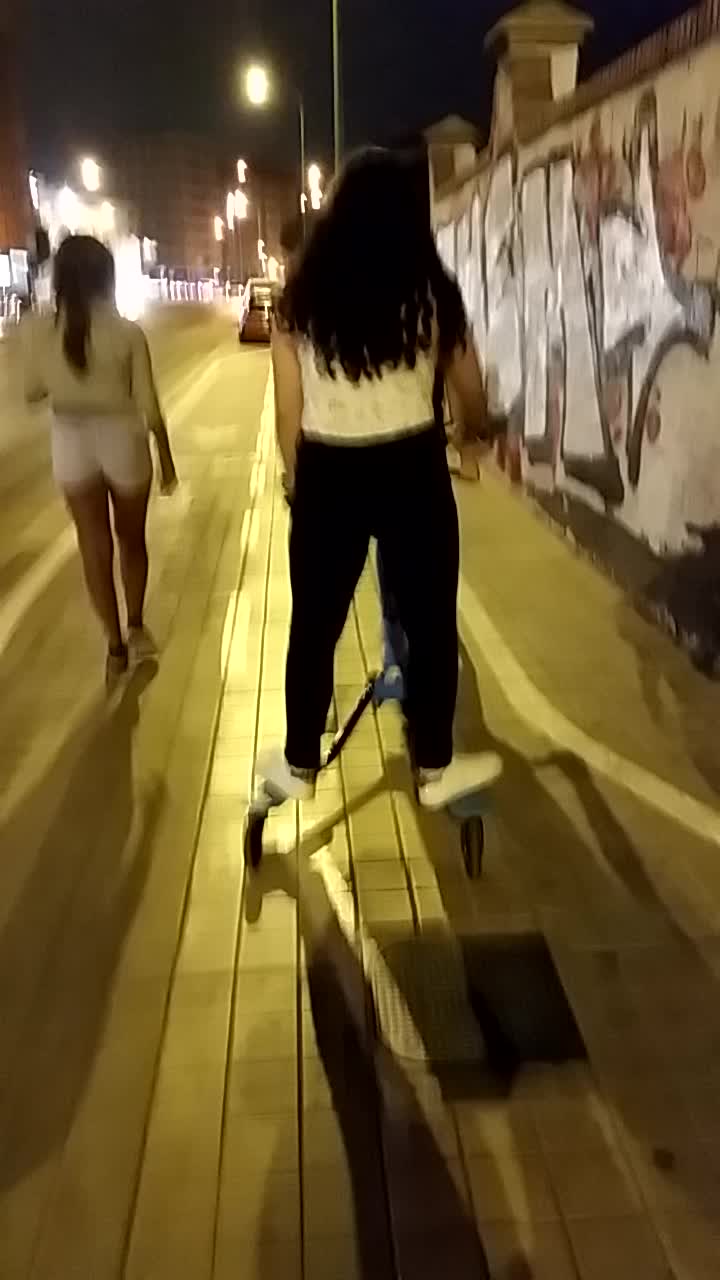The image depicts a night scene on a street illuminated by streetlights, where two individuals can be seen. The focus is on a person standing on a unique, tricycle-like scooter with a V-shaped platform of two small rear wheels and one front wheel, controlled by handlebars. This person is dressed in low white sneakers, black pants, and a white tank top, with their long hair hanging down to mid-back. The setting includes a sidewalk lined with graffiti-covered walls and streetlights, and cars are visible in the background. To the left, another individual is walking alongside, wearing white shorts and a white shirt, also with long hair, highlighting the urban setting of this bustling street.